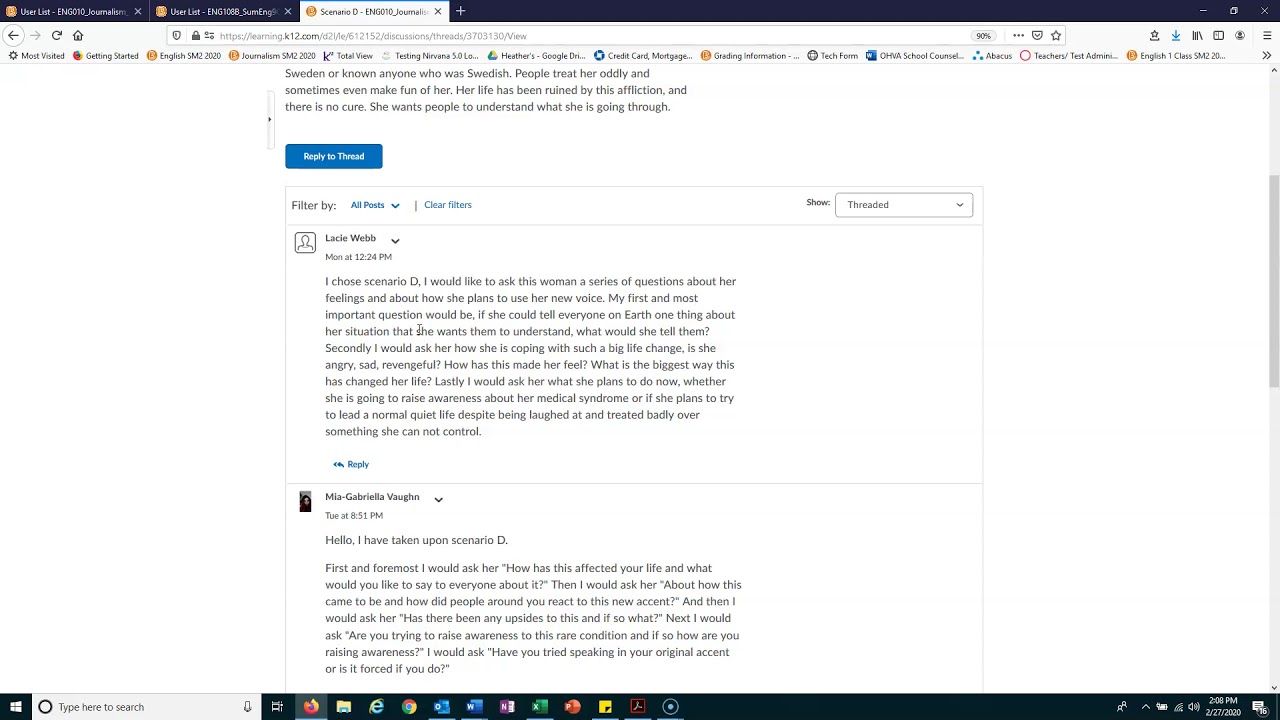The image is a screenshot of a web page with several distinct features. The web page itself contains black text and is bordered by black lines at the top and bottom. A prominent blue button is present on the page, possibly indicating a call to action or navigation element. At the bottom of the screen, there are several colored icons arranged in a row. These icons are colored red, white, green, multicolored, blue, blue, brown, green, red, yellow, black, and blue.

On the bottom left of the screen, the Windows Start button and a search magnifying glass icon are clearly visible. On the bottom right, standard system icons are displayed, including the time, battery status, internet connection indicator, and sound control.

At the top right corner of the window, there are control buttons to minimize, maximize, or exit the window. Meanwhile, the top left corner shows the browser tabs. There are three tabs in total: two tabs with black titles and one with a white background, indicating it is the currently active tab.

Overall, the screenshot captures a detailed view of a web page interface along with the surrounding browser and system elements, providing a comprehensive look at the screen's current state.